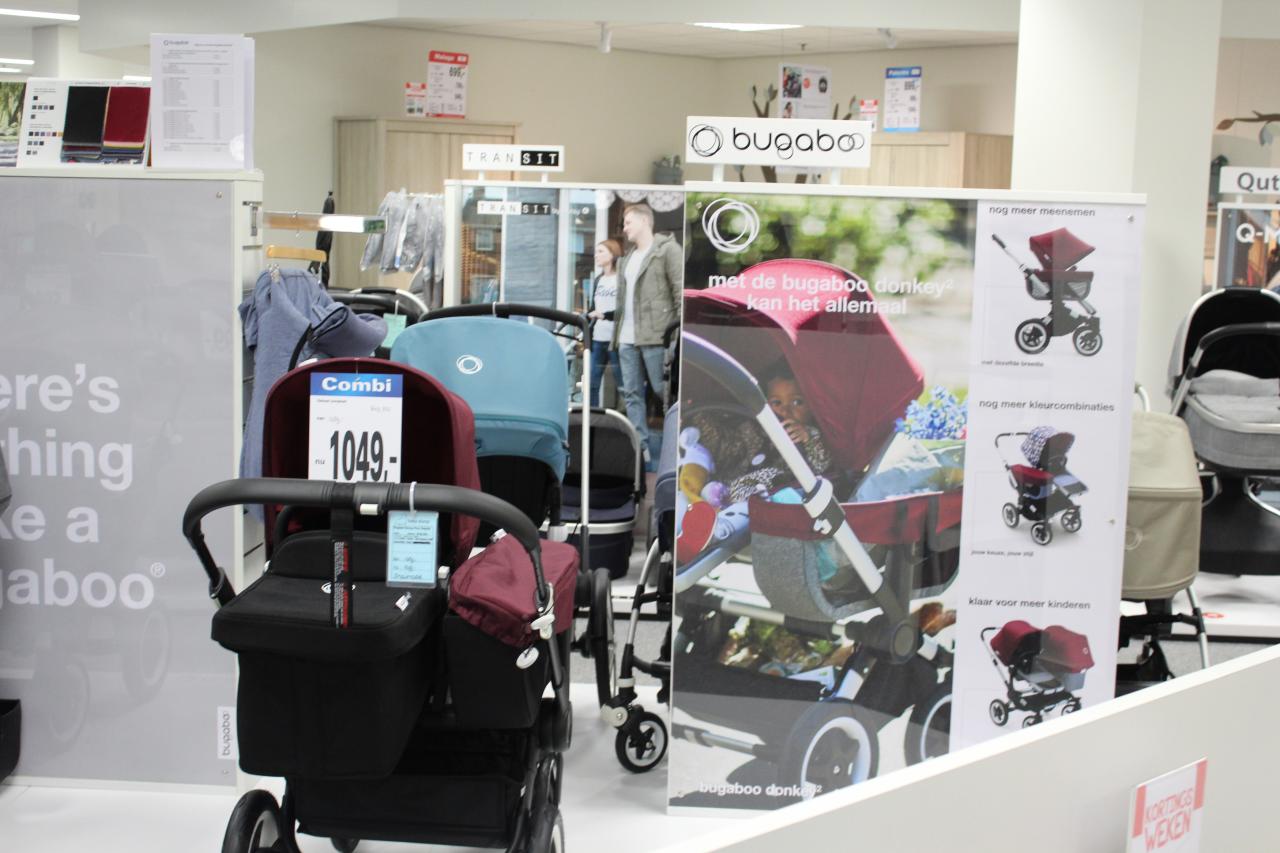The photograph depicts an interior view of a store specializing in Bugaboo baby strollers. The store features a white ceiling with recessed lighting and white walls, contributing to a clean and modern aesthetic. Centrally displayed within the room are approximately four standee displays, each providing information about the strollers, though the text is not legible due to the distance. Several strollers of varying colors are prominently showcased, including ones with maroon, light blue, and tan covers.

A notable element on the lower right section of the image is a white barrier wall, behind which stands a tall plexiglass advertisement display. This display features a prominent white sign with black writing reading "Bugaboo" and an image of a red stroller with a baby of African descent inside it. Adjacent to this, there is a price tag indicating $1,049. To the left of the advertisement, there is a partially visible gray banner with the text “there’s nothing like a Bugaboo.”

In the far background, tan-colored bookcases line the wall, further emphasizing the store’s organized layout. Additional visual details include other Bugaboo strollers and banners with images of people shopping and various clothing items. The store's detailed and varied stroller displays are the focal point, highlighting the wide assortment available for potential buyers.